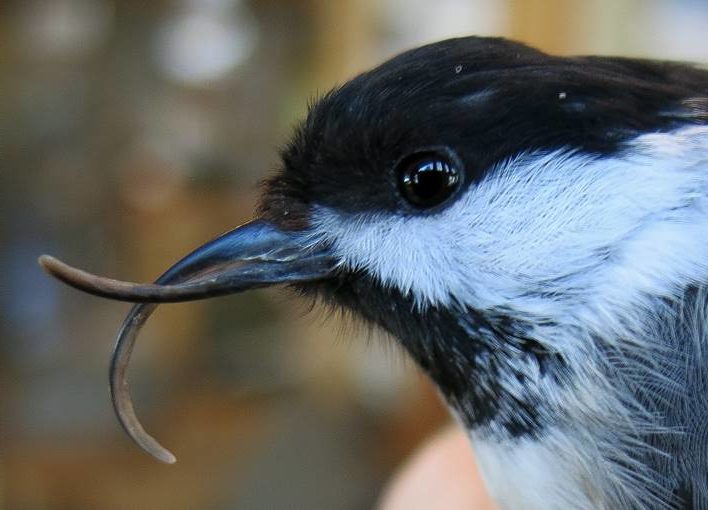This image is a highly detailed close-up of a bird, focusing primarily on its head and a small portion of its neck. The bird's head features striking black and white coloration; the top of the head is black, transitioning to white around the eye area and then black again at the throat, with some gray blending in towards the lower parts of the neck. The bird's left eye, which is black with light reflections, is prominently visible as the bird faces left, giving us a clear side profile.

The most remarkable aspect of the bird is its unusual beak. The upper beak curves downward in a pronounced arc while the lower beak curves upward, creating a distinctive C-shape where the two parts do not close or meet. This peculiar beak configuration stands out as an extraordinary feature. The background of the image is a blurred mixture of brown, light brown, orange, and white hues, which could be reflections or lights, providing a soft backdrop that enhances the focus on the bird's head.